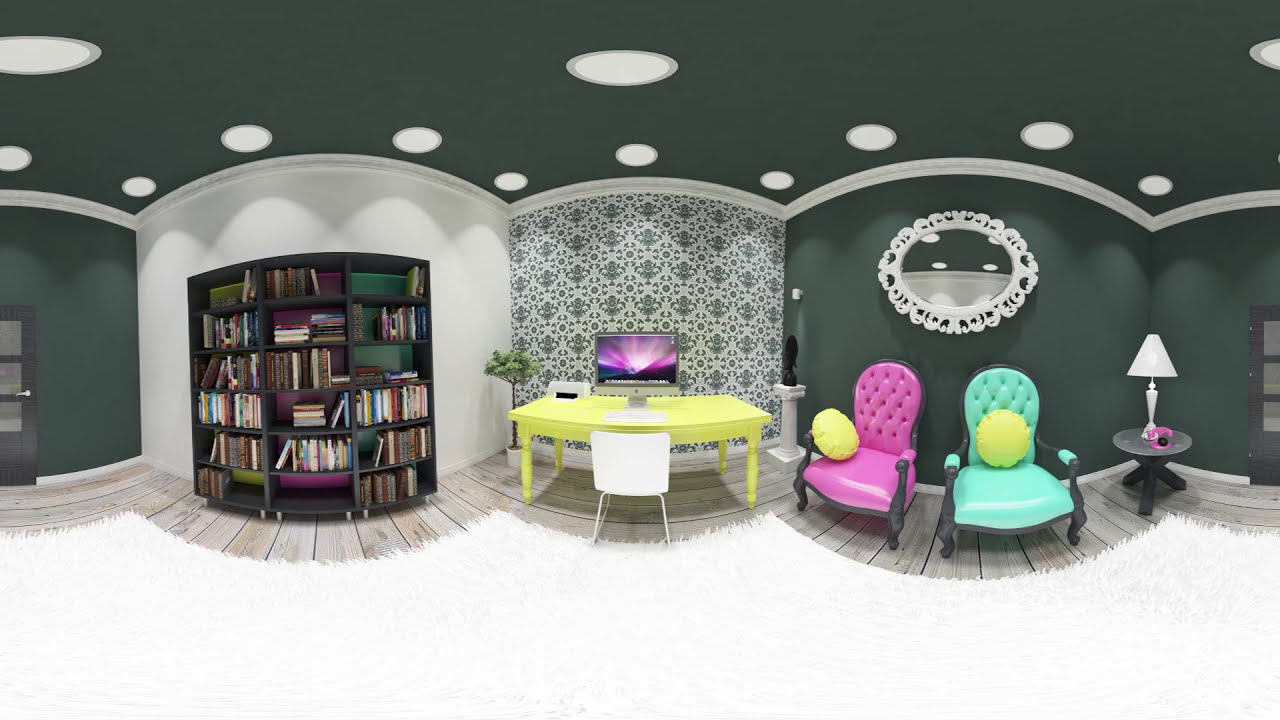The image is a highly detailed and panoramic 3D render of a room that combines various stylistic elements in greens, whites, yellows, and grays. Centrally placed in the room is a yellow desk with a desktop computer. In front of the desk, there is a soft white rug. To the right of the desk, two chairs are positioned against the wall, one pink with a yellow pillow and the other turquoise with a yellow pillow. Above them hangs a white oval mirror. Next to the turquoise chair is a small circular end table with a white lamp on it. 

On the left side of the room, there is a bookshelf filled with books, and near it stands a black door which seems to be the entrance to the room. The room's walls feature green and white colors, with the central part adorned in a patterned green and white wallpaper. The ceiling, painted in a dark green, is equipped with illuminated spotlights. The flooring consists of light gray wood, adding to the overall muted yet vibrant palette. Finally, a pedestal with a black statue is also present along the right side of the room, contributing to the eclectic decoration.